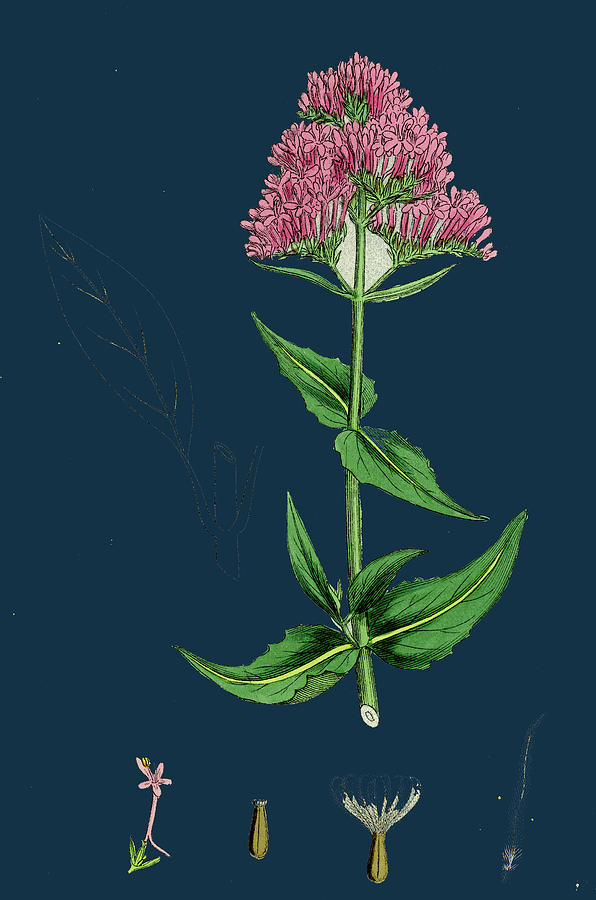This detailed, vertically aligned rectangular artistic print features a meticulous hand-drawn sketch of a flower against a solid, dark navy blue background. Dominating the center and upper portion of the image is the flower itself, with a long green stem adorned with distinctly detailed green leaves. From the bottom ascending upwards, there are two large leaves at the base, each pointing in opposite directions, followed by a set of two smaller leaves, achieving a symmetrical balance. Midway up the stem, another pair of medium-sized leaves extends outwards.

The crowning feature of the flower is its densely packed arrangement of small, delicate pink blossoms, which collectively form a rounded, almost triangular cluster interspersed with smaller green leaves. This main bloom is composed of three distinct layers of the tiny pink flowers, adding depth and texture to the illustration. 

Positioned at the bottom of the image are smaller, detailed inset drawings that further break down the flower's structure and lifecycle. On the lower left, an individual pink flower is depicted before it is fully bloomed. In the center, a detailed illustration of a seed pod is shown, and on the right, the seed pod is depicted as sprouting, with what appears to be pollen on top, highlighting its role in propagation.

The overall composition and color scheme, with the contrast of vibrant green and pink against a deep navy background, evoke a sense of summertime vibrancy and botanical beauty, possibly reminiscent of a blooming garden.